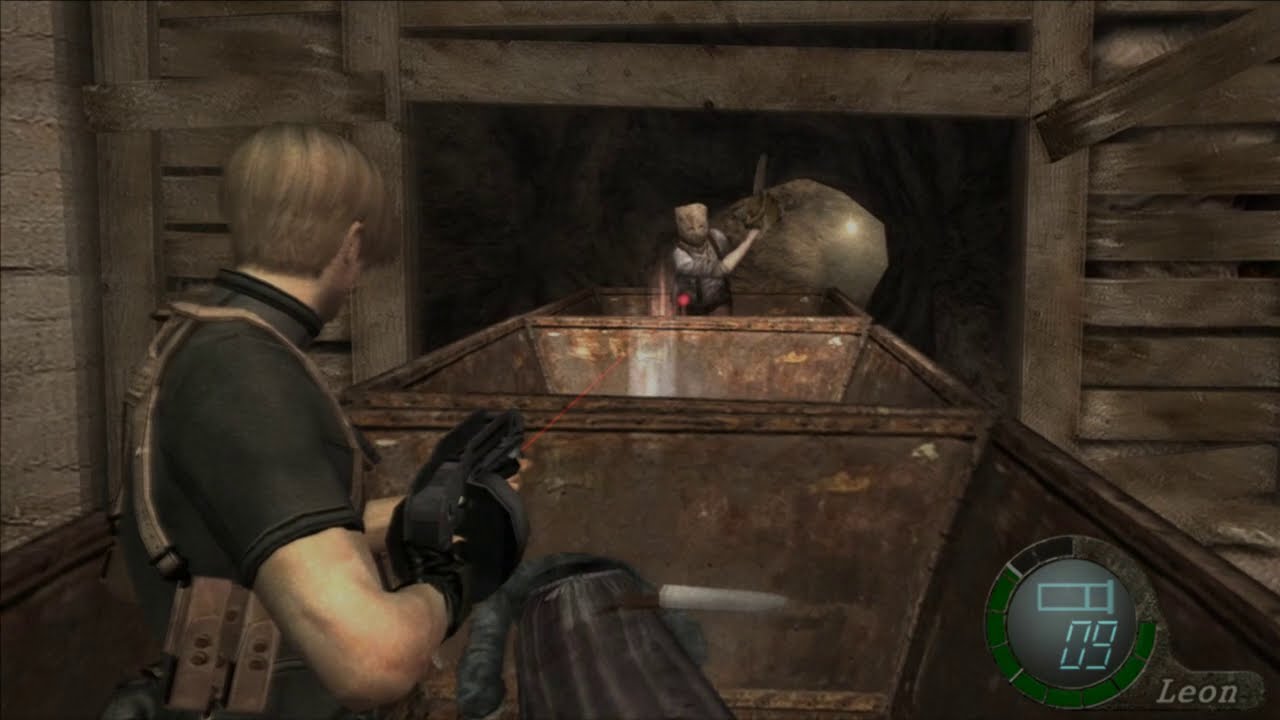In this computer-generated image from the video game "Resident Evil," we see a detailed scene set within a mining shaft or tunnel. The environment is defined by wooden planks forming the walls and supporting the entranceway, creating an ominous, enclosed space. The central focus is on two characters engaged in what seems to be an intense confrontation. The character in the foreground, seen from an over-the-shoulder third-person perspective, has wavy blonde hair and is geared up in a black t-shirt, black gloves, and a brown bulletproof vest with a holster on his right side. Armed with a black shotgun featuring a red laser scope, he is aiming at another menacing figure in the background.

The second character, who stands near train tracks in the dimly lit tunnel, has a bag over his head and is brandishing a chainsaw menacingly. He wears suspenders and appears to be an antagonist. Near this character, there are two metal train carts, and a large, round octagon-shaped stone adds to the scene’s mysterious ambience.

Also visible in the lower right-hand corner of the image is a circular interface element displaying the numbers "0-9," next to the label "Re-Own." The overall composition suggests a tense moment of confrontation and suspense within this dark, wooden tunnel.